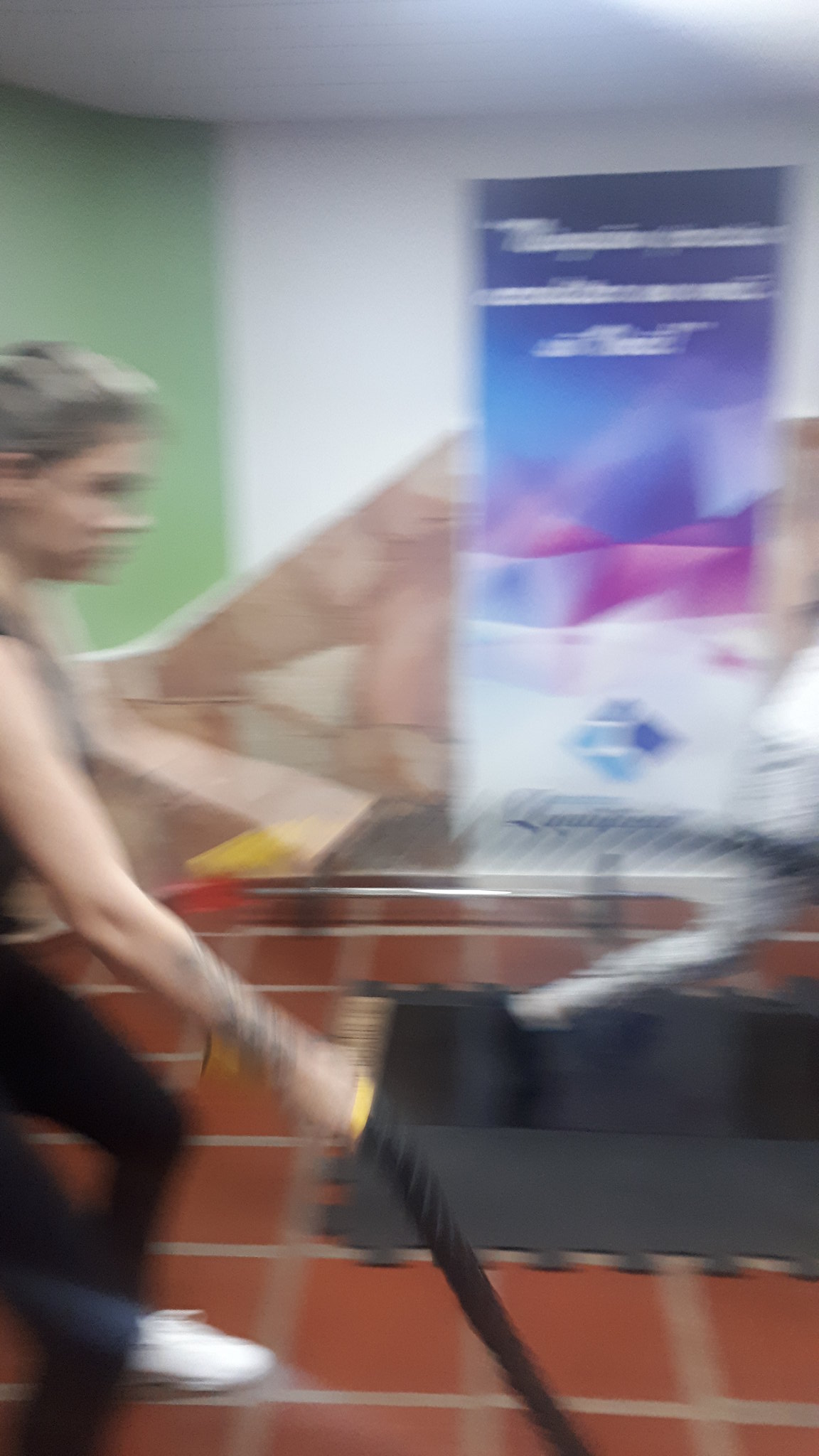A blurry, out-of-focus image captures a woman in a gym, engaged in fitness activities. She is wearing black pants and white shoes, alongside a sleeveless shirt, and is gripping a black rope with yellow ends. A tattoo can be seen on her forearm. The background features a white wall transitioning to green on the left. A large, eye-catching blue poster with white text gradually shifts in color to pink-purple, then white at the bottom with a blue diamond shape. Nearby, a machine with a black base and a white component curving right and left is visible. In the corner of the image, a yellow object is present.